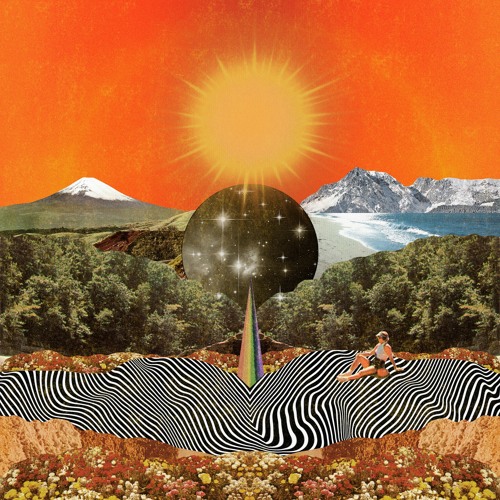The image is a vividly detailed and surreal piece of artwork, potentially an album cover. Dominating the red sky is a bright yellow sun, positioned at the top center, where it casts a halo effect. Beneath the sun to the left and right are two distinct snow-capped mountains – one greenish-grey with a white peak and the other brownish-black, also capped with snow, overlooking a beach with blue waves lapping against golden sand.

In the middle of the scene, nestled between the mountains and below the sun, is a smaller circular object resembling a galaxy, filled with a black space-like sky and sprinkled with stars. From the center of this galaxy, a rainbow arcs downward, ending in an area filled with black and white wavy lines that create an optical illusion, resting on a foundation that appears to be soil or dirt.

A human figure, possibly a woman, is relaxed and leaning back on these black and white squiggly patterns, reminiscent of lounging on a beach towel. Trees are rising towards the sun on the far left side of the image, adding to the mix of natural elements. The overall composition is psychedelic and layered, with the vibrant details and disparate landscapes merging into a distinctive, almost dreamlike scene.